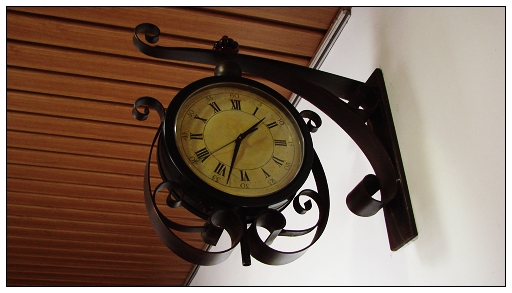This is a detailed color photograph of a vintage wall clock mounted sideways on a white wall. The clock is secured by a decorative black metal bracket that extends over a walkway, reminiscent of Victorian wrought iron work, with intricate curls and flourishes. The clock itself features a weathered, yellowed face, suggesting significant age. Its numbers are displayed in black Roman numerals. The current time showing on the clock is 1:33. Visible in the background is a ceiling constructed from hardwood planks, spaced approximately half an inch apart, adding to the rustic ambiance of the setting.